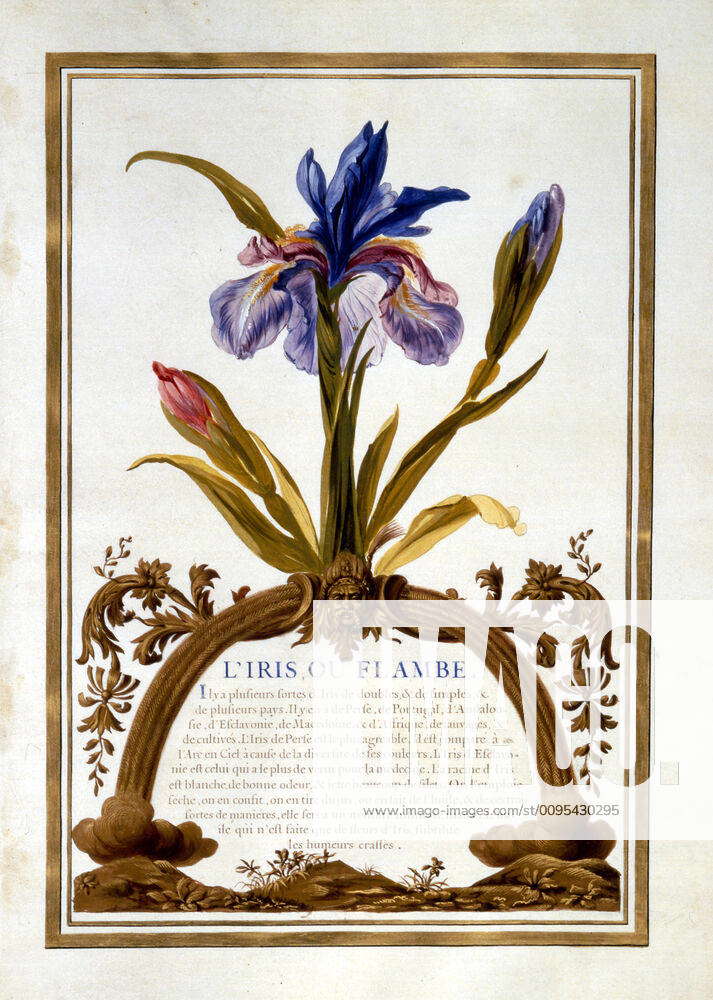The image showcases a detailed painting featuring three flowers against a white background with a sophisticated gold-border design. At the forefront is a prominent blue and purple iris, partially in bloom and accompanied by a yet-to-bloom pink bud and another upcoming blue bud. The flowers exhibit a mix of green foliage, some appearing fresh while others show signs of yellowing and decay. These flowers sprout from a double root system, intricately intertwined with an iron structure that boasts a small, ornately detailed face embedded within. The base of this structure mimics dirt and grassy terrain, adding to the naturalistic setting. Notably, the image bears a watermark reading "Imago" and a website link. There are also inscriptions in French, presumably naming the artwork as "Lyra's Iris of Flambert."